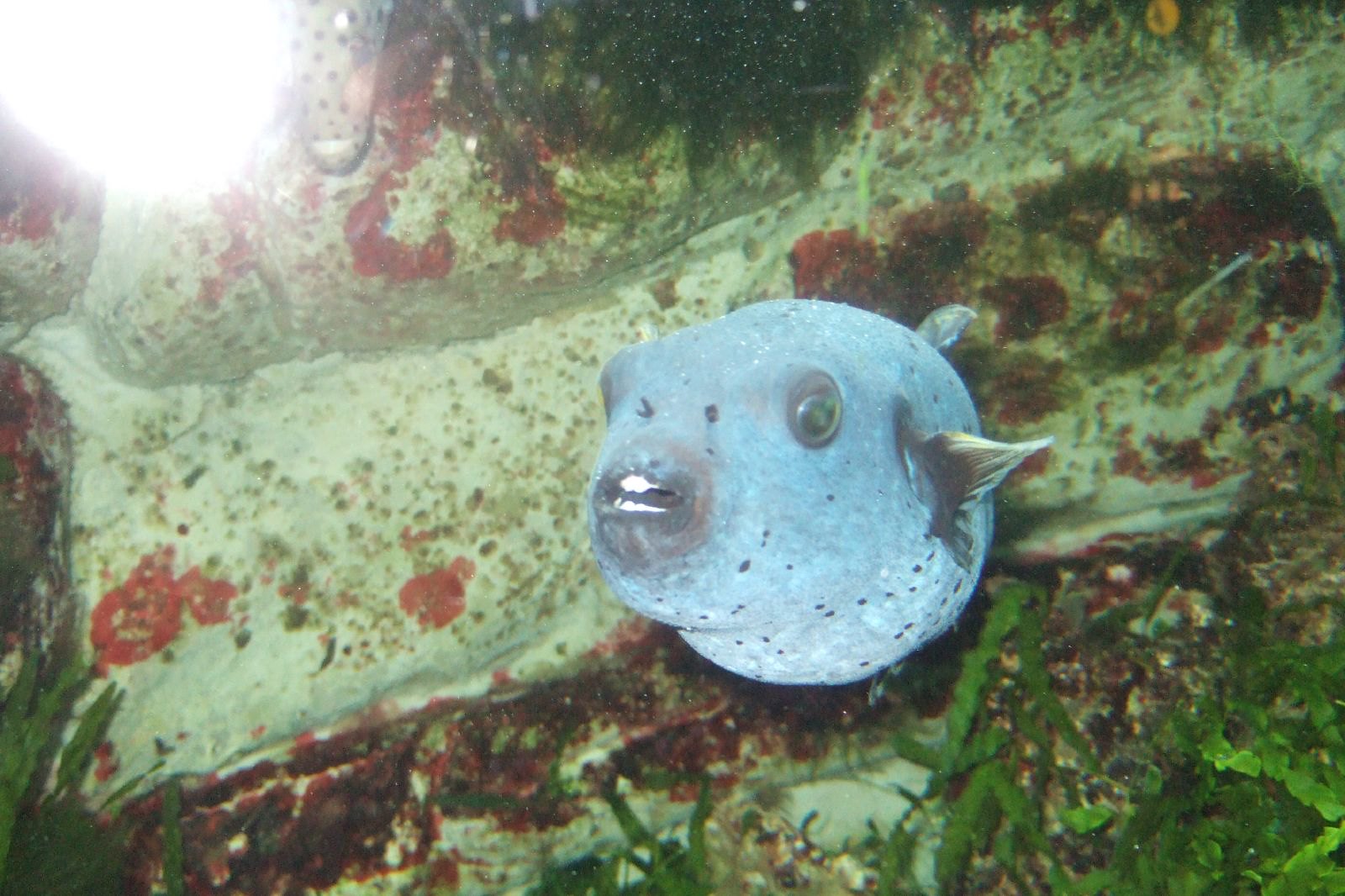In this detailed underwater photograph, a large, round fish, most likely a black spotted puffer fish, dominates the foreground. The fish is light blue with a slight bluish gray tint and intricate black spots adorning the lower part of its body. Its eyes are bright green, and its mouth is outlined in black, giving the illusion of having teeth, with its lips prominently featured. The fins are black-tipped with a touch of yellow. The fish appears to be swimming in what seems like an aquarium, as suggested by the surrounding elements—there's a backdrop resembling a wall and a noticeable glare indicative of glass. Green seaweed and algae flourish at the bottom of the scene, complemented by red seaweed and a white log-like structure adding to the aquatic ambiance. The overall setting conveys an underwater realm, with a hint of sunlight filtering through the top left, bathing the scene in a serene glow.